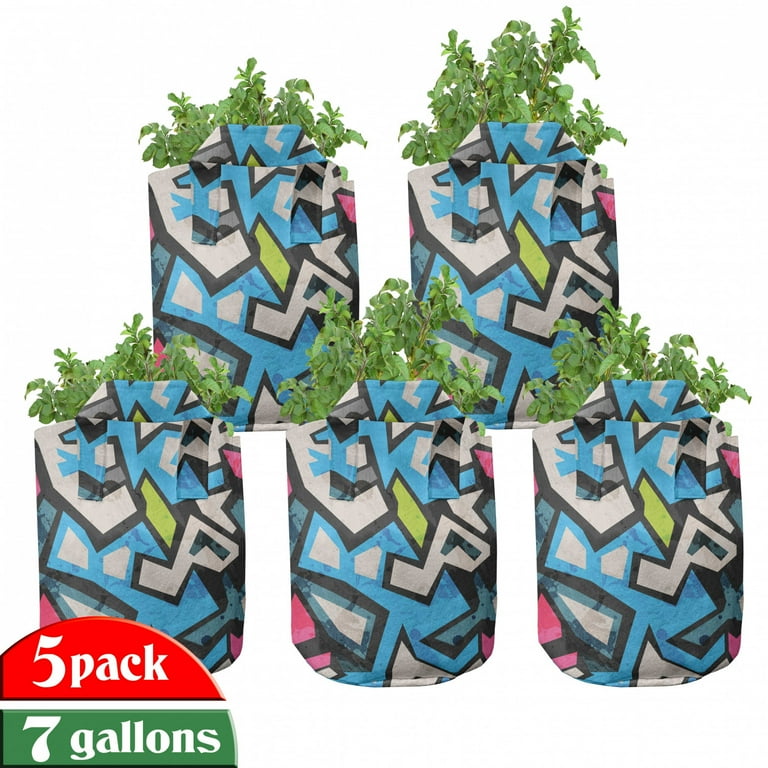The image is an advertisement showcasing five colorful bags, each designed to hold plants. These bags, wrapped in an abstract graffiti artwork of blue, silver, lime green, pink, and red sections with thick black outlines, feature green leaves or flowers sprouting from each one. The bags are arranged in two rows: two bags on the top row and three on the bottom, all set against a completely white background. In the bottom left corner of the image, there is a red semicircle with "five pack" written in white letters, and below that, a green rectangle with "seven gallons" also written in white letters. The overall aesthetic of the image is vibrant and eye-catching, though the exact purpose of the bags remains somewhat ambiguous.